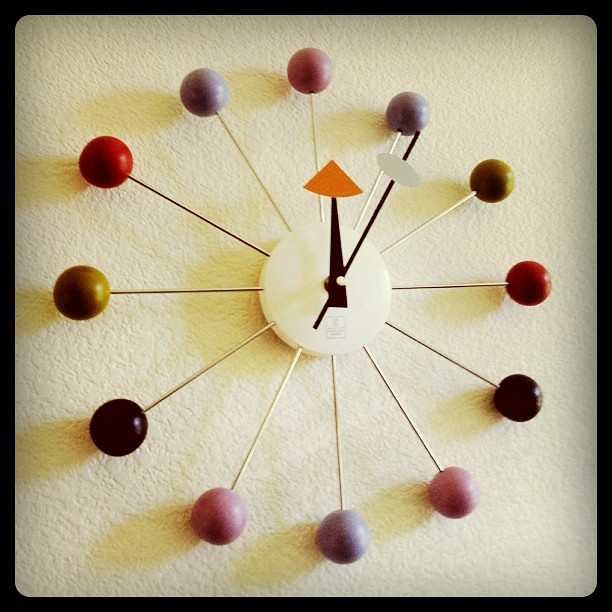This image showcases a distinctive clock design mounted on a textured surface, likely a wall. The clock features a central white disc that serves as the base for its unique hands and radiating elements. Sturdy, thick wires extend outward from the disc, each terminating in colorful balls or marbles, adding a playful and artistic flair. The hour hand is marked by a reddish triangle, while the minute hand is distinguished by a gray oval, enhancing their visibility and aesthetic appeal. The overall setup suggests a mid-century modern or abstract style, blending functionality with artistic expression.